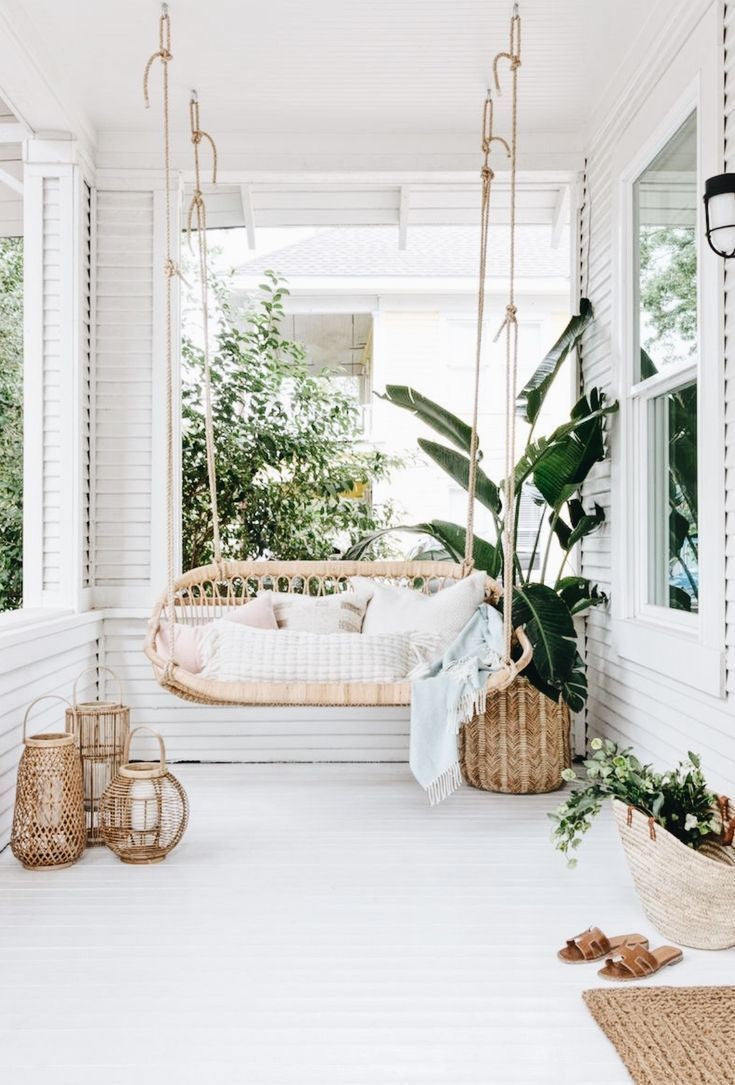The image depicts a picturesque, white front porch bathed in bright daylight. The porch features a charming wicker swing suspended from the ceiling, adorned with various cushions and a blue-edged fringe throw. To the left of the swing, three wicker lanterns, likely housing candles, add to the cozy ambiance. Behind the swing, a tropical plant in a wicker pot contributes to the verdant setting. On the right side, below a window, a wicker mat is neatly placed with a pair of flip-flops and a bag filled with leaves. The clean white wooden slats of the porch floor and ceiling frame this tranquil space, with the greenery of trees visible in the background, enhancing the overall serene and inviting atmosphere.